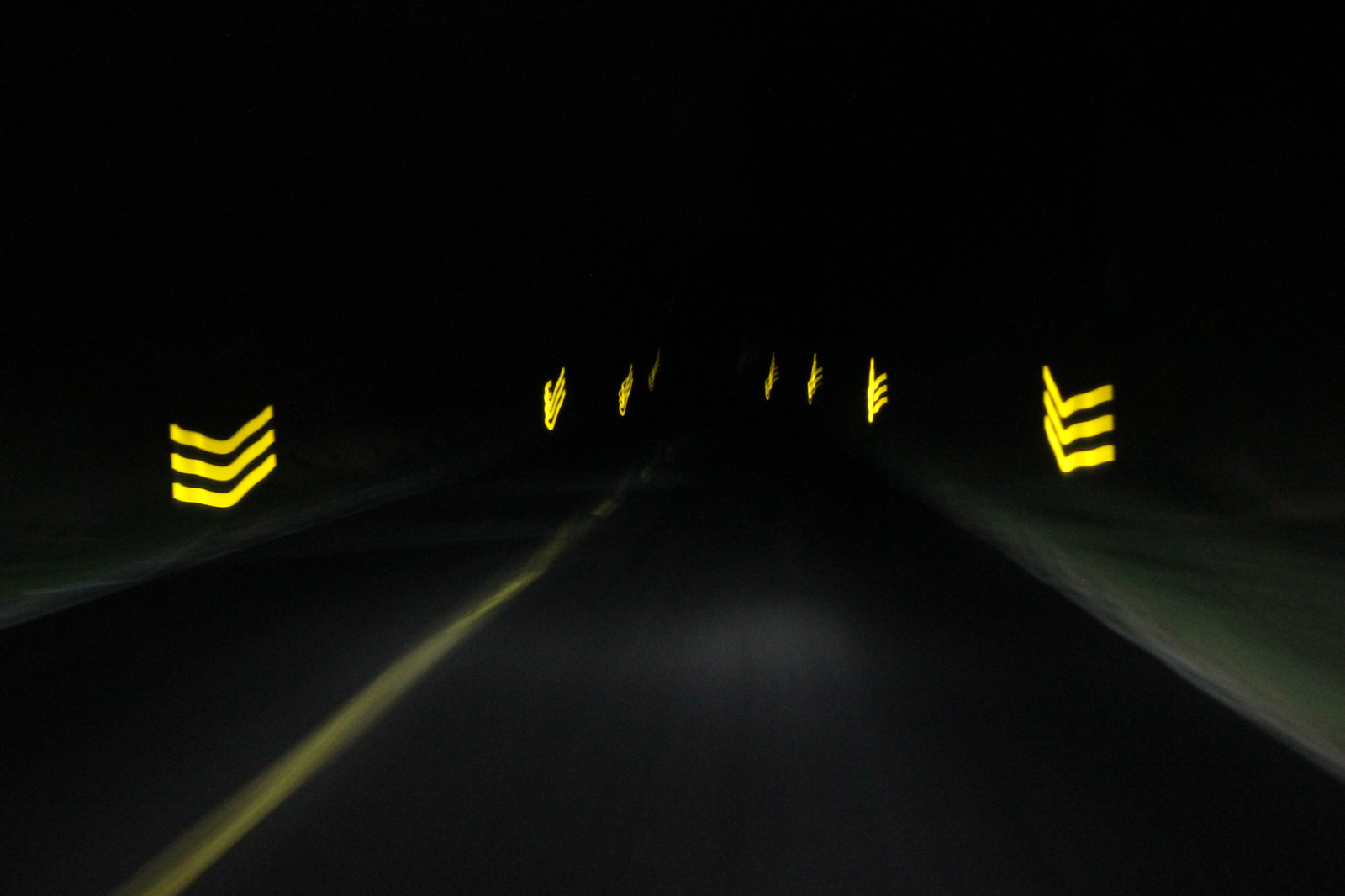This image showcases a computer-generated scene of a two-lane highway, each lane presumably facilitating traffic in opposite directions. The representation is predominantly black, creating a stark contrast with the vivid yellow line that marks the division between the lanes. Adding a unique element to the scene, eight floating downward-pointing triangles—reminiscent of military rank insignias—are positioned symmetrically on either side of the highway, facing towards each other. Despite its modern appearance, the exact timeframe of the image's creation is uncertain. The surreal, almost futuristic visual elements suggest it could be from a recent digital artwork or a slightly older computer-generated design.